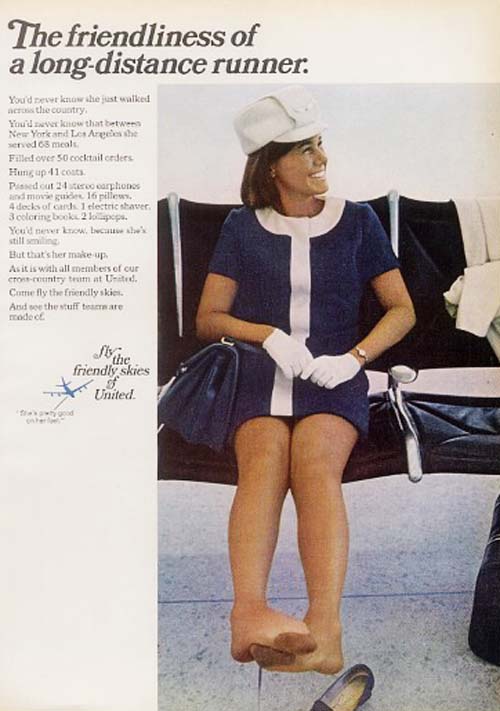This image is a vintage magazine page, likely from an in-flight publication by United Airlines, featuring an old advertisement for stewardess employment. The page has aged, with the whites taking on a brownish tint, as if it were scanned from an old, worn copy. Dominating the right side of the page is an elegantly dressed, dark-skinned woman in a classic 1960s-1970s flight attendant uniform. She wears a sky-blue dress with a white stripe down the middle, white gloves, a white hat, and pantyhose. Her high heels rest on the concrete floor beneath her, and she sits atop a black bench with a large blue purse by her side. She smiles brightly, revealing her teeth, and gazes to the right, seemingly towards someone off-camera. The title at the top of the page reads, "The Friendliness of a Long-Distance Runner." Along the left side, an article introduces her with, "You’d never know she just walked across the country," and continues to describe her duties between New York and Los Angeles, mentioning she served 65 meals, filled over 50 cocktail orders, and hung up 41 coats, among other tasks before the text fades and becomes difficult to read. This ad encapsulates the theme of "Fly the Friendly Skies of United."